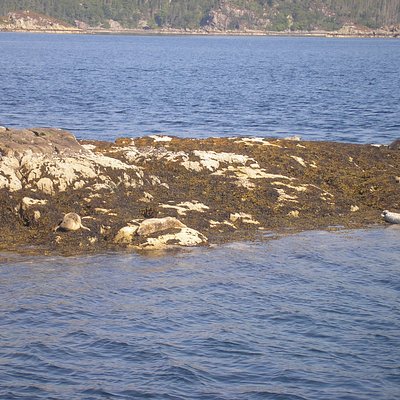The image captures a tranquil nature scene primarily focused on a horizontal strip of rocky and earthy land set in a larger body of blue water. At the bottom of the image, the water shows gentle ripples leading up to the strip of land which runs horizontally across the center. This land strip is a mix of dark brown soil with patches of white rocks, occasionally interspersed with greenish hues suggesting vegetation or algae. The scene suggests the strip might be a miniature island or a protrusion of land within a lake or river. Above this strip, a larger expanse of water stretches towards the horizon where, at the top of the image, there is a distant landmass. This distant land features dense tree cover and rocky surfaces, potentially indicating a forested area with a rocky shoreline. No text is present in the image, which evokes a serene, untouched natural setting, reminiscent of a scene one might encounter in a nature photograph.